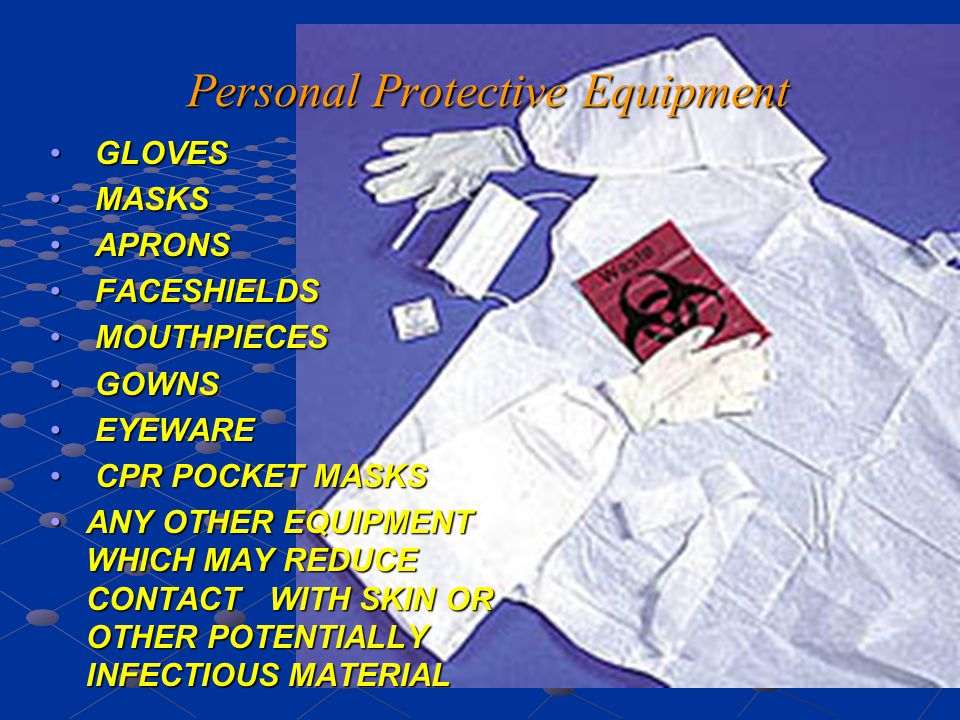The image showcases personal protective equipment against a dark blue solid background. At the top center, in orange Roman italicized font, the title reads "PERSONAL PROTECTIVE EQUIPMENT." On the left side, there's a left-aligned bullet point list in blue with item names in uppercase yellow Arial font, including: "GLOVES," "MASKS," "APRONS," "FACE SHIELDS," "MOUTHPIECES," "GOWNS," "EYEWEAR," "CPR POCKET MASKS," and "ANY OTHER EQUIPMENT WHICH MAY REDUCE CONTACT WITH SKIN OR OTHER POTENTIALLY INFECTIOUS MATERIAL." On the right side of the image are visual examples of the mentioned equipment. Visible are white gloves, a white mask, a white apron, and a small red book labeled "WASTE" with a black symbol. The image serves as a detailed guide for identifying various personal protective equipment used to minimize exposure to hazardous materials.